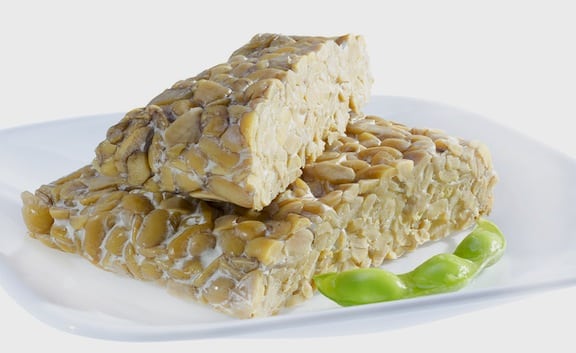The image shows a rectangular white plate set on a white surface, featuring two stacked peanut crispy cakes. The top cake is a smaller, halved version of the bottom one, revealing a cross-section where the peanuts are visibly bound together by a white cream. The tan-colored cakes, appearing hard and intricately cut, are detailed with peanuts. Accompanying the cakes is a vibrant green pea pod placed prominently in front, adding a splash of color. The scene is bright and clear, likely an indoor setting, capturing a simple yet appealing food presentation.